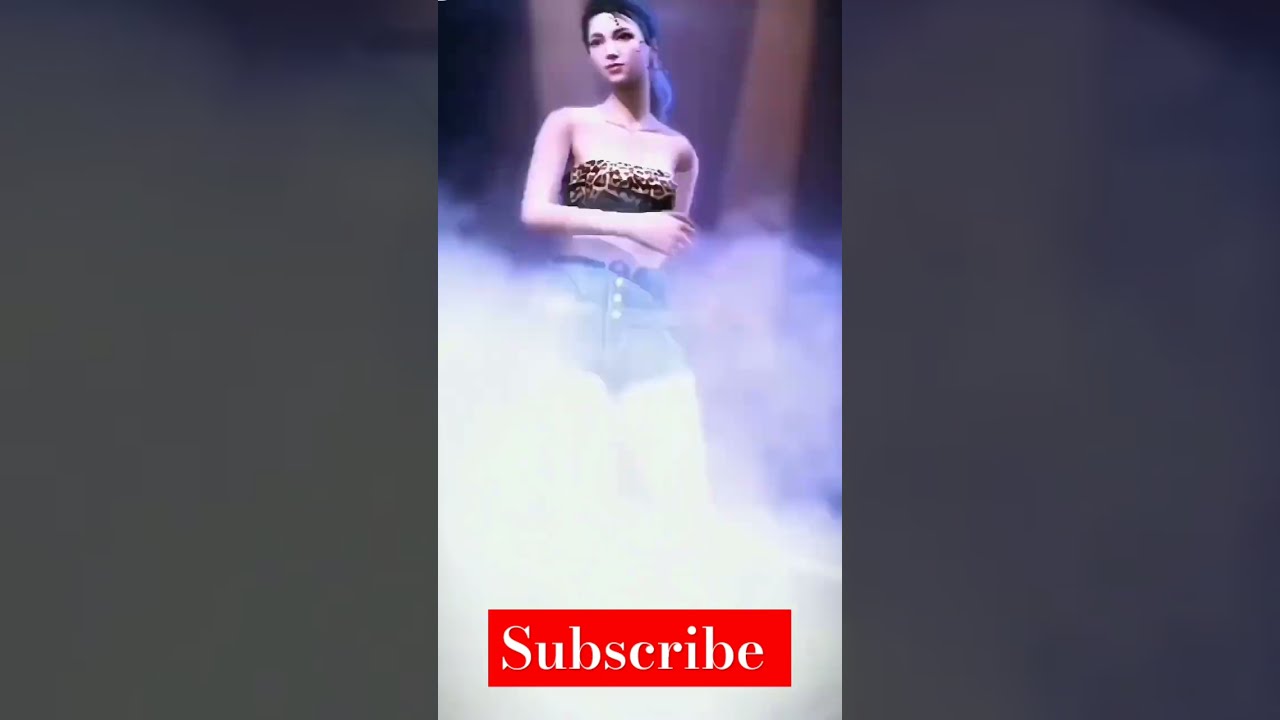The image is horizontally divided into three segments, with the left and right panels filled with black rectangles. At the center is a vertically aligned, digitally-rendered figure of a white woman, likely an avatar from a video game. She has dark hair and dark eyebrows, and is wearing a strapless, cheetah-print bandeau top that exposes her midriff. Her left arm is folded across her body. She is also wearing high-waisted jeans with three buttons and a belt. Additionally, there is some smoke or fog visible at the bottom of the picture, partially obscuring her jeans and leg area. At the bottom of the image is a red bar with white serif text that reads "subscribe," suggesting this is a screenshot from a YouTube video, possibly related to gaming content.